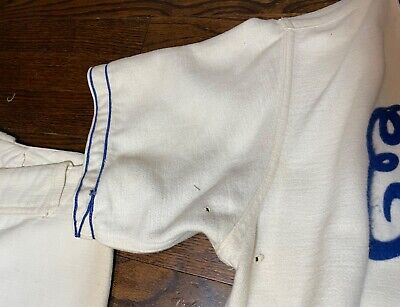The image depicts a highly zoomed-in view of a dark brown wooden surface, possibly a table, chair, or counter, though the exact object is indiscernible. The wood features longitudinal planks with varying shades, including darker spots and lighter specks, enhancing its textured appearance. Positioned prominently in the frame is the sleeve of a shirt, predominantly white with blue lines and partial blue script text, revealing only an "E" in cursive. Adjacent to the sleeve, there is another fabric, though heavily folded and close-up, making its identity uncertain. A hint of what might be a belt loop is also visible, adding to the ambiguity of this piece of clothing.